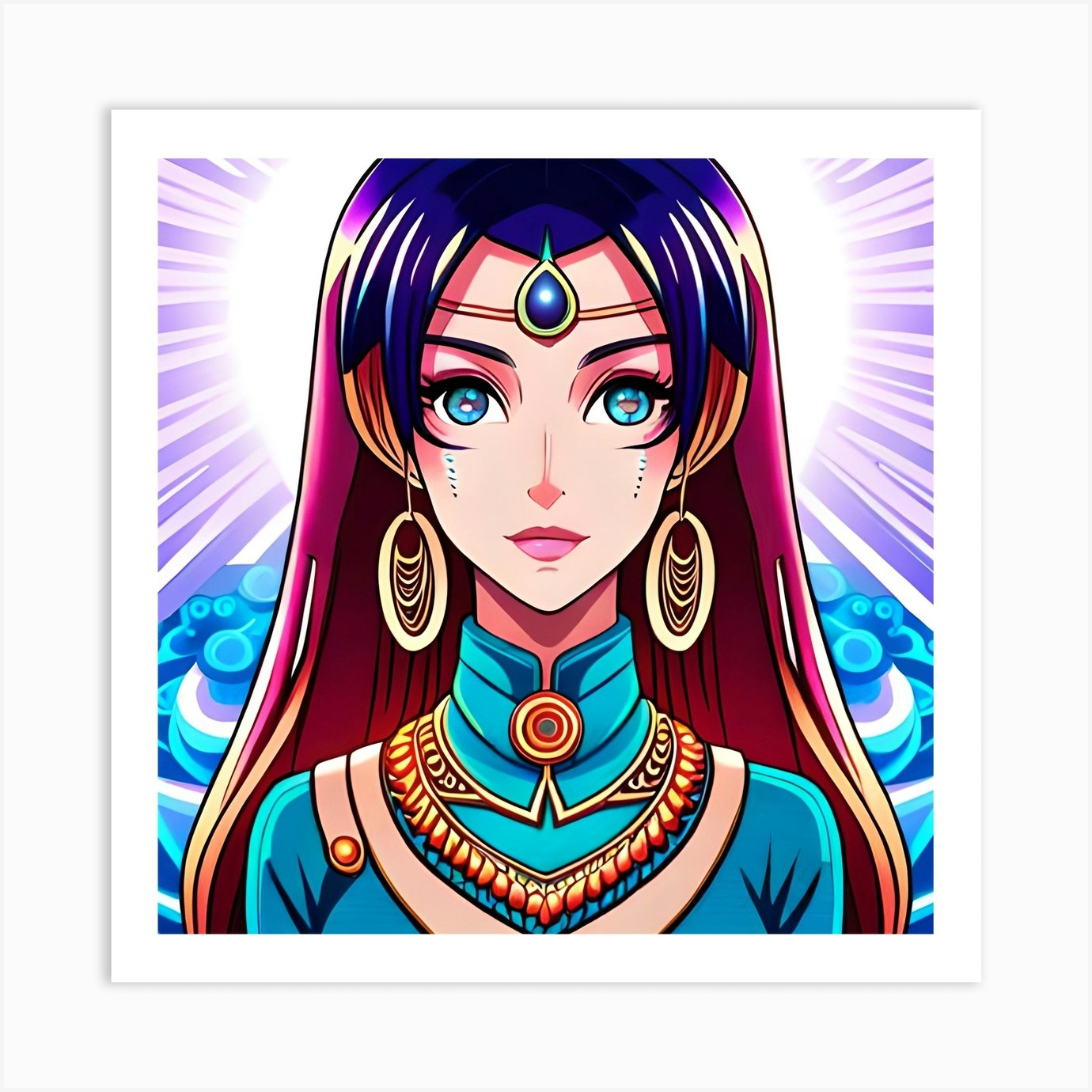The digital art piece depicts an anime-style girl with striking blue eyes. Her multicolored hair transitions from blue at the bangs, to a fuchsia-to-red gradient, and finally to orange and yellow at the tips. She adorns a distinctive blue gem with a golden setting on her forehead and wears large, gold hoop earrings. The girl is dressed in a blue top with a high collar, complemented by a gold-trimmed V-neck and small gold leaf-shaped gems around the neckline. Behind her head, a purple sunburst emanates, adding a dramatic backdrop to the image. The art is framed with a white border, and another inner lighter white border, encapsulating the detailed composition.